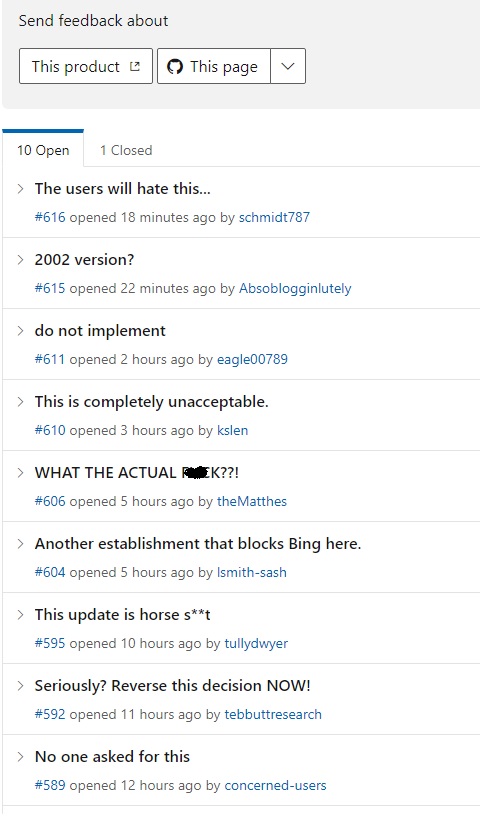The image is a vertically oriented rectangle set against a predominantly white background. At the very top, a thick light purple ribbon spans the width of the screen, bearing the text "Send feedback about" in black. Beneath this ribbon, there are two white buttons side by side. The left button features the text "This product" in navy blue, while the right button displays "This page" accompanied by a drop-down arrow.

Below these buttons, on a white backdrop, the text "10 open 1 closed" is displayed, with the "10 open" section highlighted by a bright blue bar above it. Following this, a vertical list of feedback entries is presented. Each entry includes a subject title in bold black text, an entry number in bright blue, and a timestamp indicating how long ago it was opened, along with the user's name in bright blue.

The first entry reads "The users will hate this..." and is identified as feedback number 616, opened 18 minutes ago by Schmidt 787. The second entry, titled "2002 version," was posted 22 minutes ago by the user abso blogging loots, identified as entry number 615. The third entry, "Do not implement," was entered two hours ago by eagles 00789. The fourth entry, "This is completely unacceptable," was opened three hours ago by KSL EN. The list continues in this manner, featuring various feedback entries and complaints.